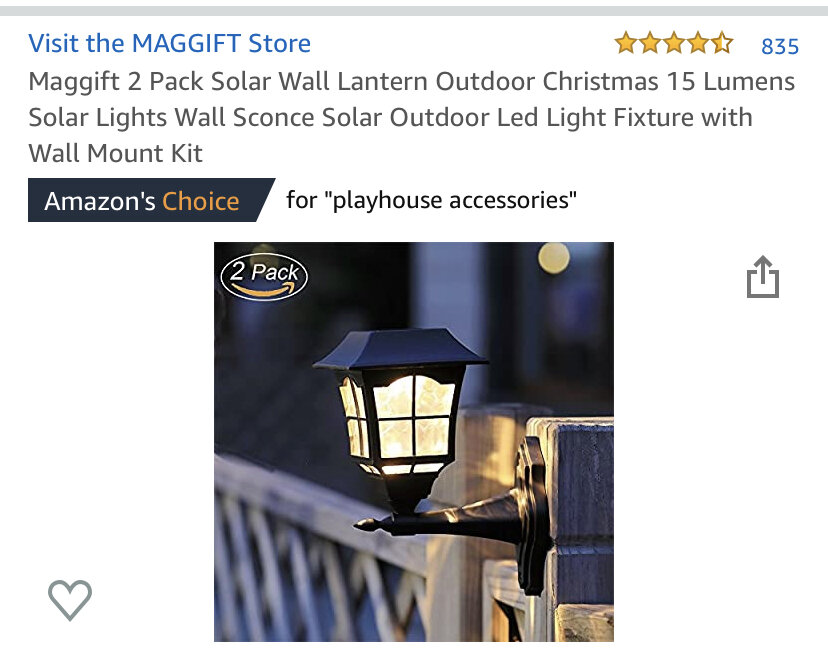**Detailed Caption:**

Screenshot of an Amazon listing showcasing a "Magic Two-Pack Solar Wall Lantern Outdoor Christmas 15-Lumen Solar Lights Wall Sconce." The item has a high rating of 4.5 out of 5 stars, based on 835 reviews. This product is endorsed by Amazon, featuring an "Amazon's Choice" badge, specifically recommended for "Playhouse Accessories". 

In the middle of the listing, there is a prominent image of one of the wall-mounted lanterns. The lantern is affixed to a fence post or patio beam, and it extends upwards. The scene appears to be photographed at night as the lantern emits a bright light, illuminating the surrounding area. 

Above the lantern image, on the top left corner, it is indicated that this is a "Two-Pack" with a small Amazon arrow logo beneath it. The background of the listing is white, with most of the text in black. The phrases "Visit the Magic Store" and "835" are highlighted in blue, while the star ratings are depicted in yellow. There is also a small grey heart symbol located at the bottom left corner, likely for adding the item to a wishlist.